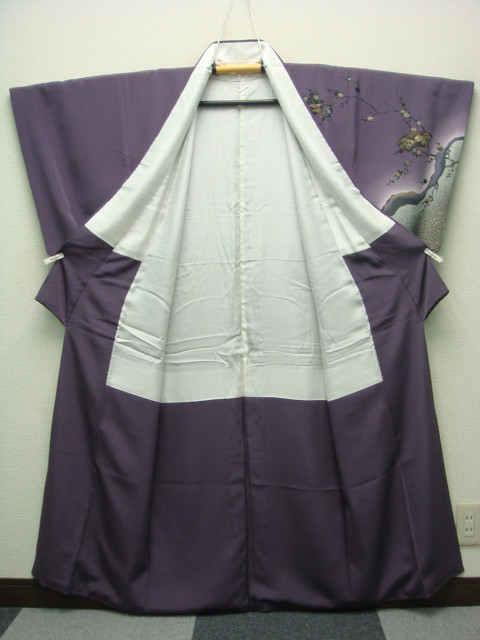The image depicts an indoor scene with a multi-colored tile floor in shades of green, white, gray, and black. Against the white wall in the background, which has a brown border along the bottom edge, hangs a piece of fabric that appears to be a dark purple and white curtain or robe. The fabric is suspended from a wooden rod or hanger, positioned centrally in the image. In the upper right corner of the fabric, delicate tree branches adorned with small, whitish flowers can be seen. Additionally, an electrical socket with two plugs is visible at the bottom right of the image. There are no texts, people, or other noticeable objects in the image, and the scene is well-lit, enhancing the clarity of the visual details.